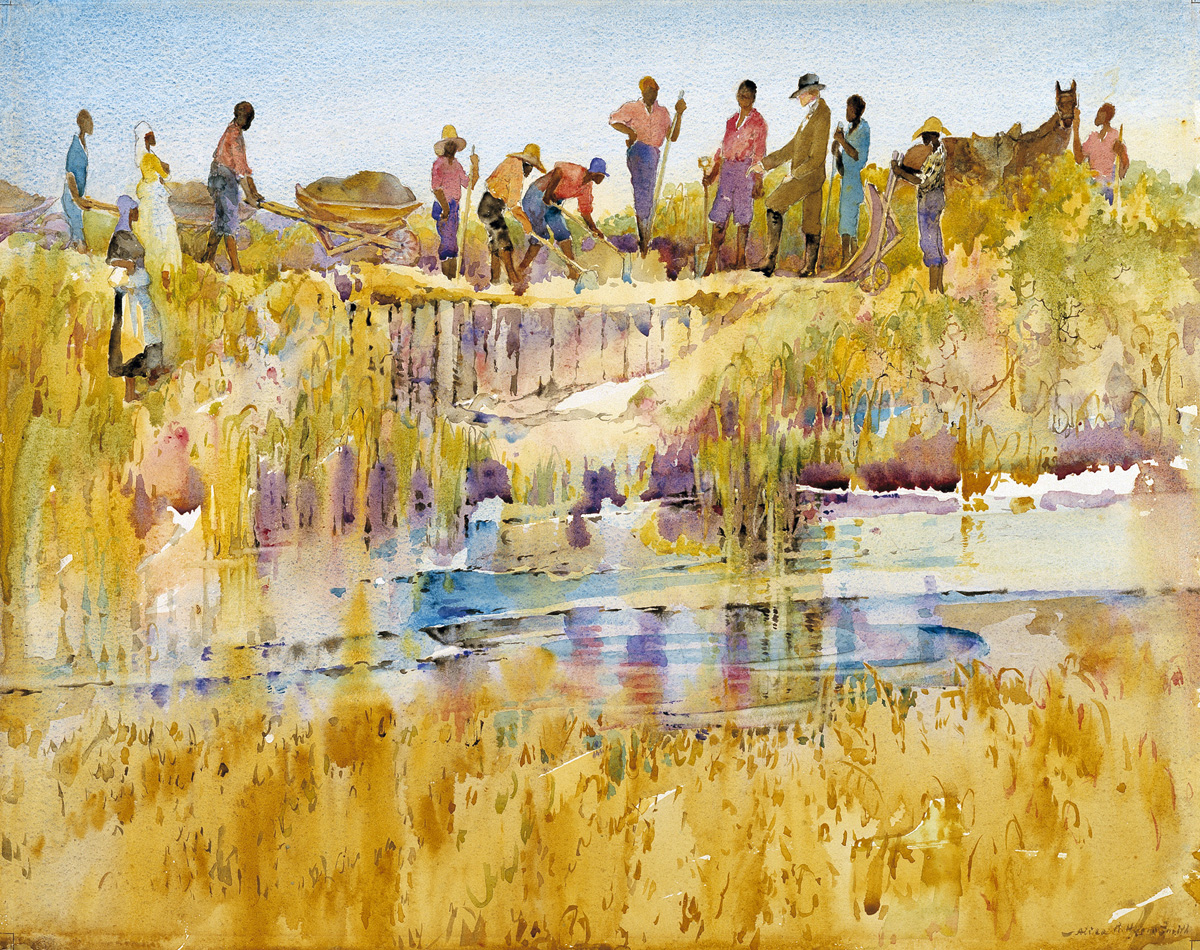The painting is a vibrant watercolor that captures an outdoor scene of people laboring in a field. In the lower third of the image, a stretch of yellow-brown grasses or hay signifies a dry environment. Above this, a stream, depicted with blue and purple hues, flows gently, bordered by a shoreline exhibiting similar colors. The focal point includes several darker-skinned individuals diligently working, dressed in colorful garments such as pink, purple, blue, and orange shirts and pants. They are engaged in tasks that involve hoes, shovels, and a wheelbarrow overflowing with soil. Adding to the scene's vibrancy, they wear straw hats and have their sleeves rolled up. On the right side, a lighter-skinned individual, presumably the landowner, stands observing. She is adorned in a brown suit, black riding boots, and a black hat. Nearby, a brown horse stands, accompanied by another figure. The background transitions into another field and is enveloped by a light blue sky. The artwork masterfully blends these elements to depict an energetic farming scene by a peaceful stream.